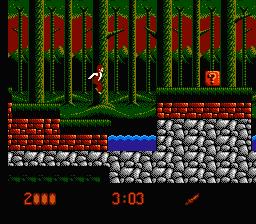In this vibrant video game scene, a small character is navigating a horizontal platform environment, moving from left to right across various textured terrains. The game screen prominently showcases multiple texture layers, starting with a rocky base at the bottom, followed by a layer of red bricks, and then a lively green grass layer. Interspersed between these layers are water-filled holes, adding a dynamic challenge to the gameplay.

Amidst this adventurous setting, the character is captured mid-jump above the green grass terrain. Towering above this scene on the highest platform is a red box adorned with a conspicuous question mark, inviting curiosity and interaction.

The background further enhances the visual experience with gently undulating green hills and scattered green trees set against a striking red sky, creating a surreal and whimsical atmosphere. At the bottom of the screen, a black bar displays the time as "23:03," adding a sense of urgency to the gameplay. The overall composition is a rich and engaging snapshot of the game's intricate design and vibrant aesthetic.